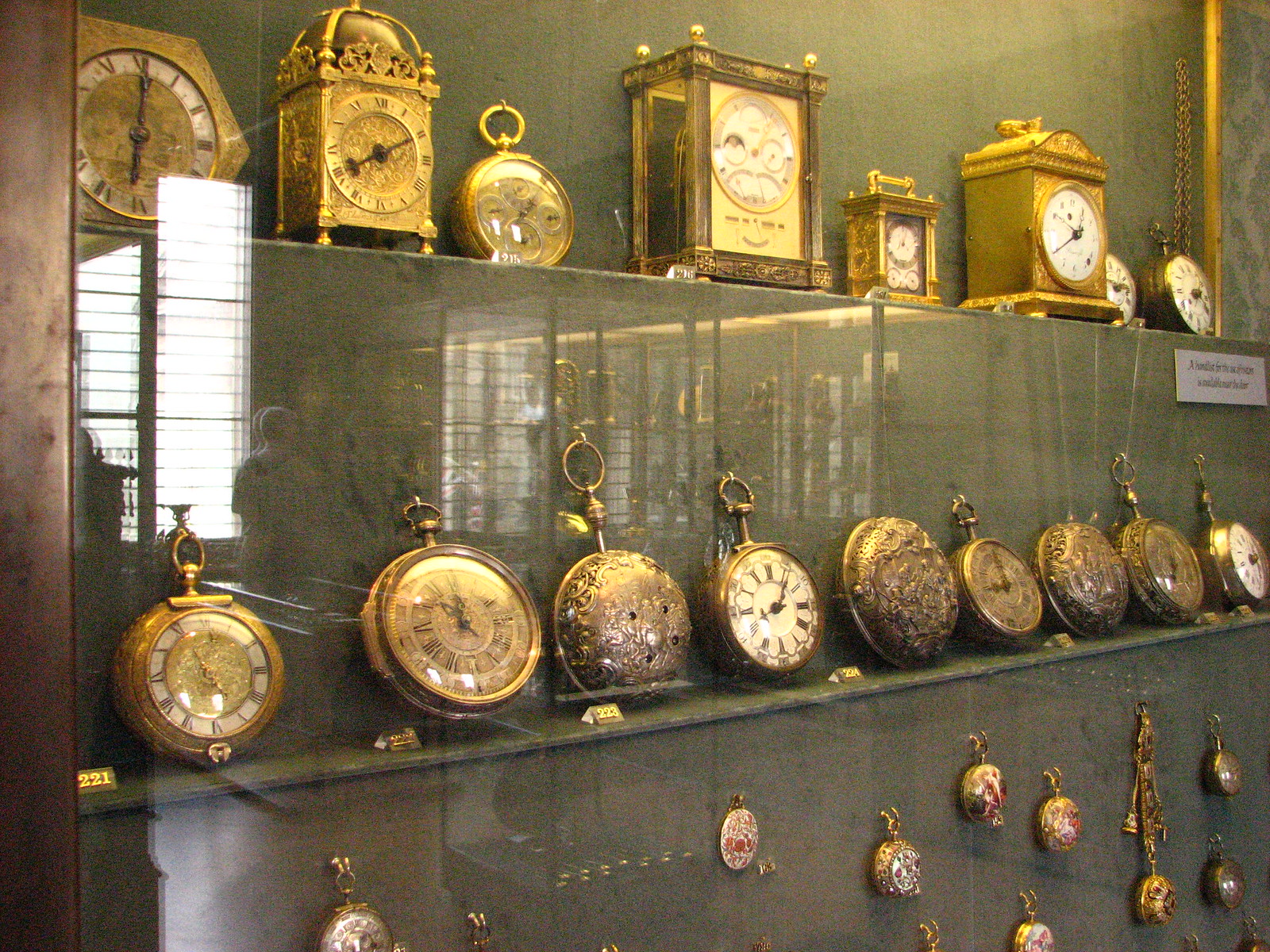The image depicts an elegant glass display case with multiple shelves, showcasing an array of antique and decorative timepieces against a dark green backdrop. The top shelf features large, square gold-plated clocks adorned with Roman numerals, accompanied by a few round hanging clocks with both dark brown casings and white backgrounds, prominently displaying their black clock hands. The middle shelf is dedicated entirely to circular hanging clocks, some embellished with front plates, exuding a sense of timeless craftsmanship. The bottom shelf is a collection of exquisite pocket watches and smaller timepieces, many detailed with ornate gold chains in dark goldish and bronzy hues. Reflections on the glass front reveal the surrounding museum environment, including glimpses of people and windows, adding depth to the overall setting. On the right side of the display case, a less noticeable steel placard with writing contributes to the historical ambiance of the scene.